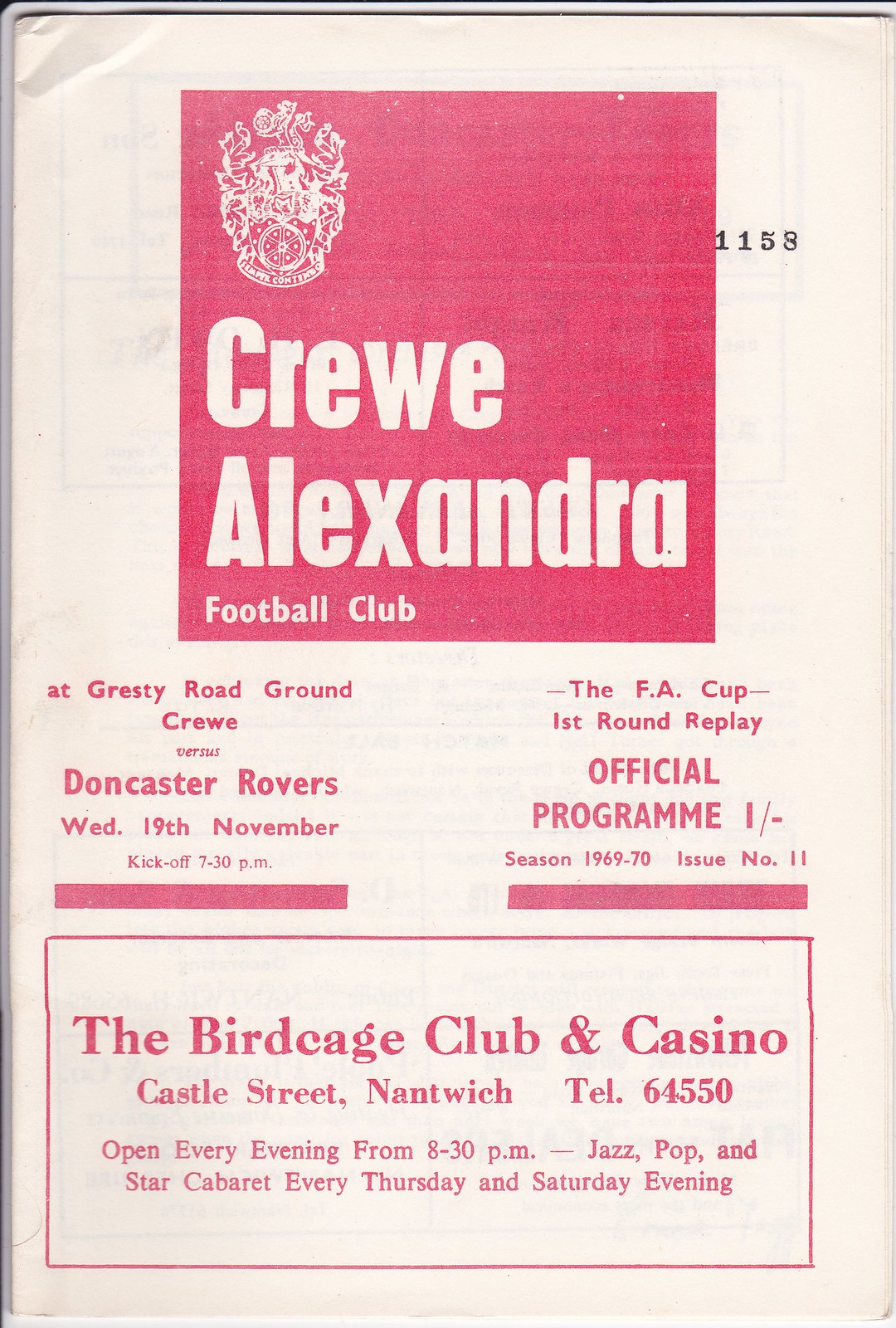This image is a close-up photograph of the cover of an official soccer program from the 1969-70 season. The program has a crisp white background, slightly crinkled at the upper left corner. Dominating the middle upper section is a large light red square with bold white text that reads "Crewe Alexandra Football Club." Beneath this, reverting to a white background with light red text, it details "At Gresty Road Ground, Crewe vs. Doncaster Rovers, Wednesday, 19th November, kickoff 7.30pm." Explicitly, the program is for "The FA Cup First Round Replay Official Program, Season 1969-70." At the very bottom, in light red lettering, an advertisement reads "The Birdcage Club and Casino, Castle Street, Nantwich, Telephone 64550," noting it is open every evening from 8.30pm and features Jazz, Pop, Insta, Cabaret every Thursday and Saturday evening.